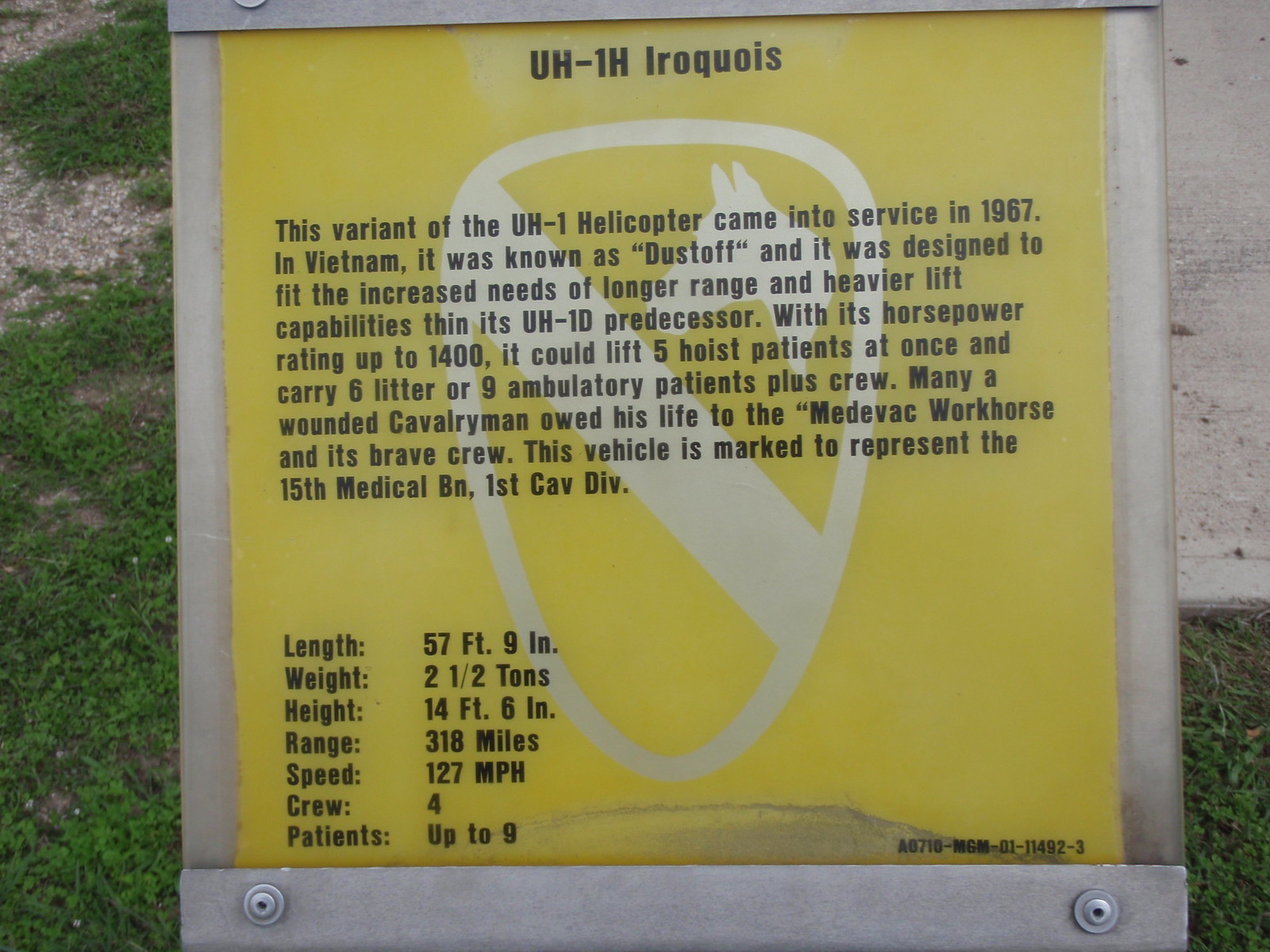The image shows an outdoor photograph of an informative plaque encased in plexiglass and bolted to a metal frame. The predominantly yellow plaque features a silver shield with a silver stripe diagonally and the head of a horse in the upper right corner. The top of the sign reads "UH-1H Iroquois." The plaque details that this variant of the UH-1 helicopter came into service in 1967 during the Vietnam War and was known as "Dust-Off." It was engineered to address the need for longer range and greater lift capabilities than the UH-1D predecessor. With a horsepower rating of up to 1,400, the helicopter could lift five hoist patients simultaneously and carry six litter or nine ambulatory patients plus crew. The UH-1H was a medivac workhorse and a lifesaver for many wounded cavalrymen, representing the 15th Medical BN, 1st Cavalry Division. Additional details include its length of 57 feet 9 inches, weight of 2.5 tons, height of 14 feet 6 inches, range of 318 miles, speed of 127 miles per hour, and a crew of four. In the background, there's grass and a cement surface, suggesting an outdoor display.